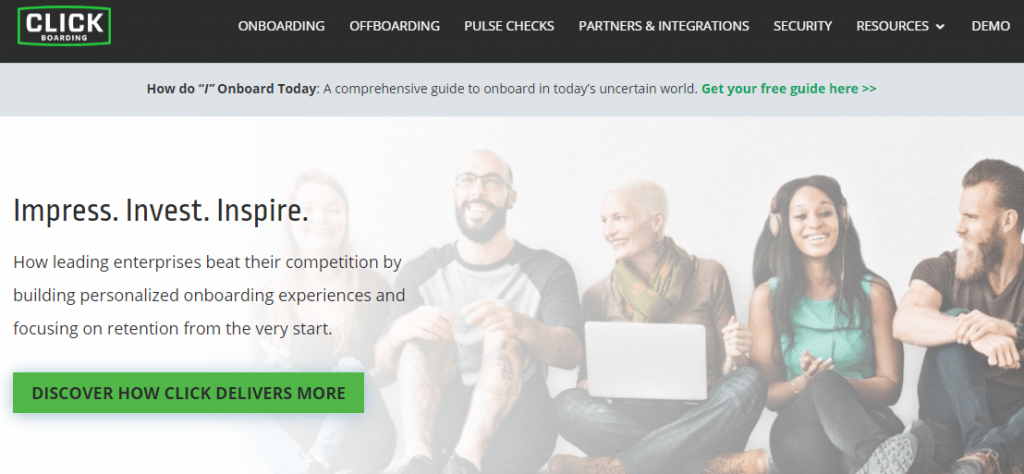The image depicts a website, potentially a mock-up, tailored for a small business. The website's top banner is entirely black, featuring a "Click" logo in white, surrounded by a green box outline. Adjacent to the logo, a list of links in white text lines the banner: "On-boarding", "Off-boarding", "Pulse Checks", "Partners and Integrations", "Security", "Resources" (with an arrow indicating a drop-down menu), and "Demo".

Beneath the banner lies a gray section proclaiming "How do I on-board today? A comprehensive guide." Adjacent to this text, a green link invites users to "Get your free guide". Directly below, a large promotional image gradually fades into transparency on its left side. The photo features a diverse group of 20-40-year-olds, both men and women, sitting together against a white wall, engaged in cheerful conversation.

The left side of this main section is headlined with "Impress, Invest, Inspire". Underneath, a descriptive text states, "How leading enterprises beat their competition by building personalized on-boarding experiences and focusing on retention from the very start." This section also includes a prominent green button with black text that reads, "Discover how Click delivers more," inviting user interaction.

Overall, the design is clean, modern, and user-friendly, reflecting the professional yet approachable ethos of a small business website.